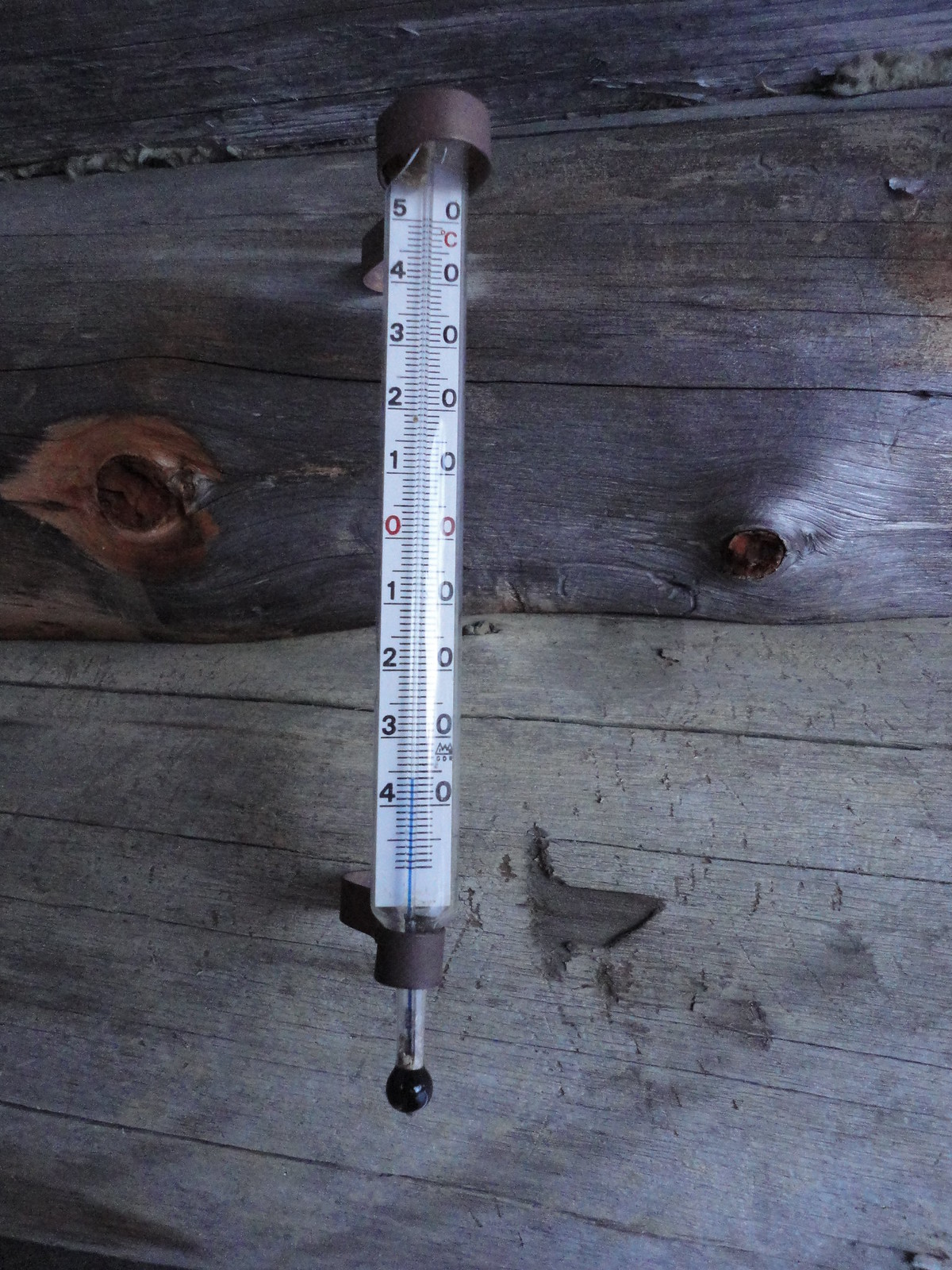A detailed photograph captures a large, barometer-like device prominently displayed against a weathered, untreated wooden wall that has a rough, gray appearance. The device is securely mounted with two metal brackets, one placed at the top and the other at the bottom, both of which are rounded to conform to the shape of the instrument. The device itself resembles an inverted thermometer and features a central vertical scale. At the top of the scale, the number 5 is clearly marked, followed sequentially by descending numbers 4, 3, 2, and 1, down to 0. Below the 0, the numbers continue in ascending order: 1, 2, 3, and 4, suggesting a symmetrical design where 0 serves as the midpoint or baseline. To the right of these numbers is a column marked exclusively with zeros, likely indicating a reference or baseline measure. Additionally, there is a small 'C' denoting Celsius temperatures. At the very bottom of the device, there is a small metal projection capped with a black plastic tip, perhaps serving as a functional or protective element. The overall setting and design create a rustic yet precise ambiance, emphasizing the device's utility in measuring environmental factors.